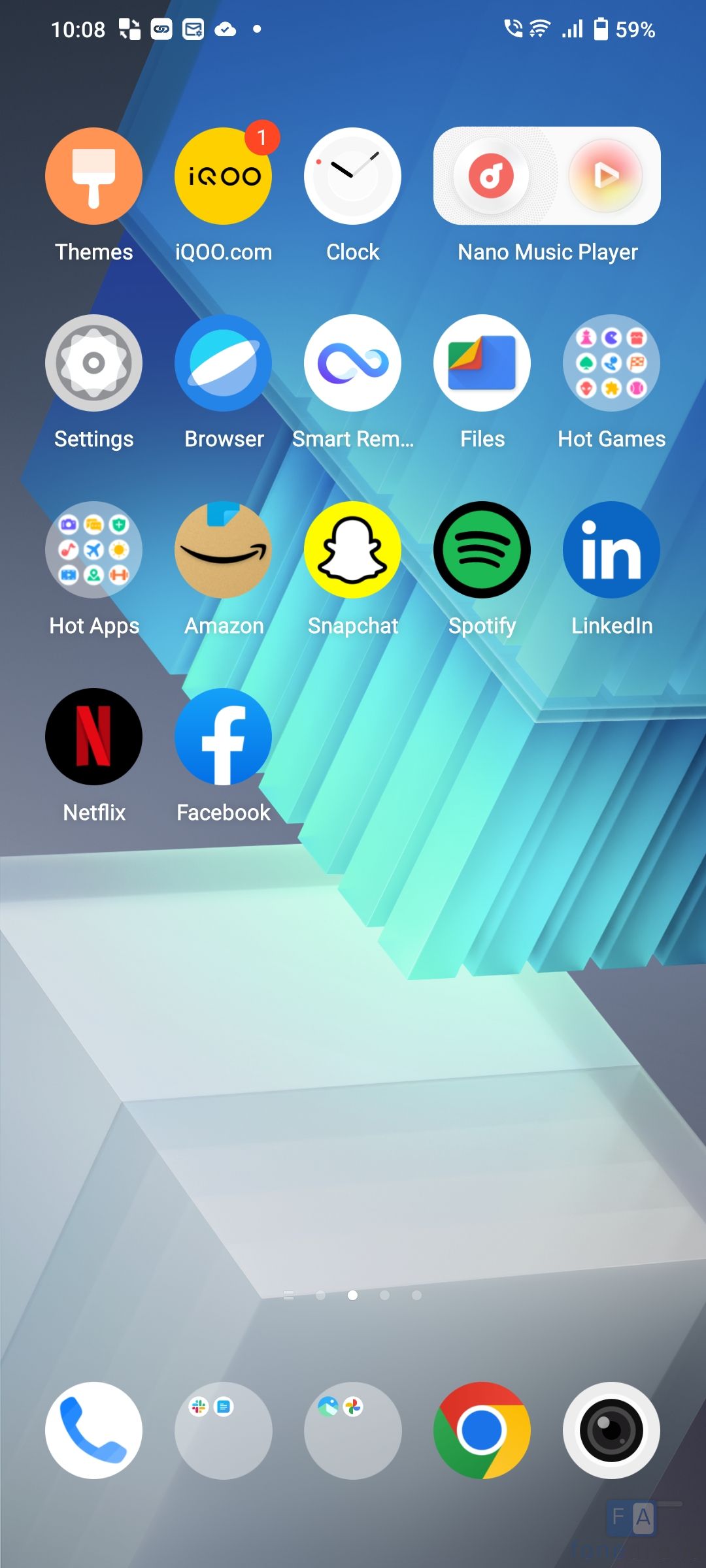This image is a screenshot of a smartphone home screen, showcasing a well-organized layout over a visually appealing abstract wallpaper. The wallpaper features gradients of light blue transitioning into gray and white geometric shapes.

**Details of the image:**
- **Time and Battery Indicator:** The top-left corner displays the current time as 10:08, while the top-right corner indicates the battery level at 59%.
- **App Layout:** The screen hosts four rows of apps, meticulously arranged:
  - **First Row:** Consists of "Themes," "IQOO.com," "Clock," and a large "Nano Music Player" button.
  - **Second Row:** Includes "Settings," "Browser," "Smart REM," "Files," and a folder named "Hot Games" containing nine icons.
  - **Third Row:** Features another folder named "Hot Apps," also containing nine icons, followed by individual apps "Amazon," "Snapchat," "Spotify," "LinkedIn," "Netflix," and "Facebook." Notably, the "IQOO.com" icon, which is yellow with a notification badge, indicating one unread notification.
  - **Bottom Row:** Displays core function icons for the phone, which include "Phone," two light gray folders with two apps each, "Google Chrome," and an additional app represented by a telephone icon.

Overall, this detailed home screen organizes essential applications and folders efficiently, ensuring quick access to frequently used functions and services.